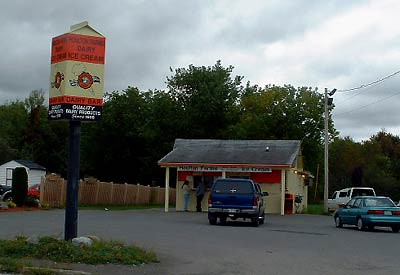This image captures a small, rustic ice cream stand resembling a tiny restaurant located in a rural, likely Midwestern setting. The stand, no larger than a shed or a small kitchen, has a brown roof and is accompanied by a wooden brown fence on the left. In front of the stand, there are two people standing by the window, indicative of a customer service interaction. The parking lot in front of the stand contains three vehicles—one directly in front and two more on the right. To the left of the stand, there is a prominent sign mounted on a large black pole, designed to look like an orange and white milk carton, with text at the bottom in black with white letters that are too small to read. The sky overhead is overcast, adding to the quiet, rural ambiance of the scene. In the background, a row of trees frames the entire setting, with power lines visible on the right side of the image.